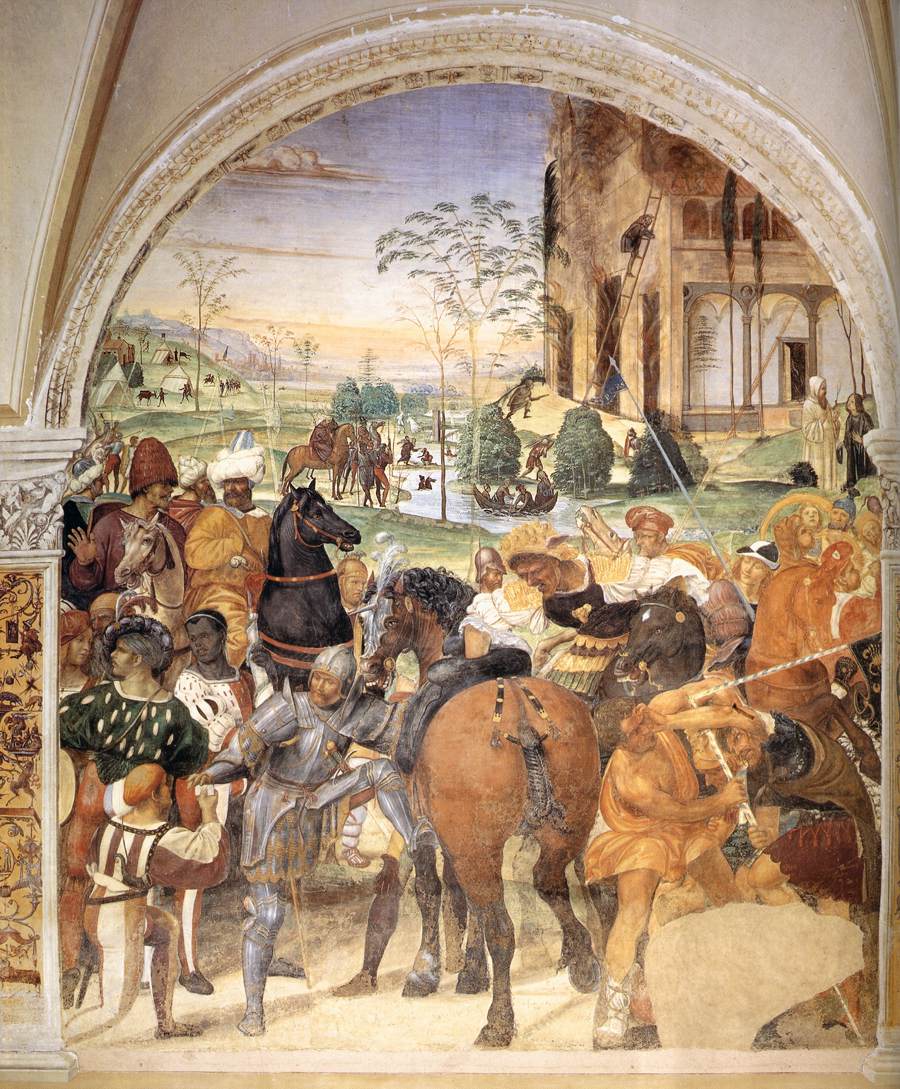This vertical rectangular painting presents a medieval scene viewed through a detailed archway that starts about halfway up and features concrete-colored moldings and patterned designs. Through the archway, one can see a bustling tableau of humans and horses set against a clear blue sky with high clouds. Dominating the foreground is a brown horse with a dark black curly mane, seemingly directed by a knight clad head-to-toe in silver armor. To the left, another knight in armor rides a black horse with a brown harness, while a mocha-colored horse stands further back with a light mocha harness. Amidst the bare dirt, people crowd around, including a short person in a dark green harlequin-like top holding the knight's hand. The knight's horse is distinguished by a metallic plate on its forehead, adorned with a silver feather. In the background, a cream-colored building can be seen, possibly near water, where some horses are positioned near a stream. Trees, shrubs, and even ladders are visible, along with a green hill dotted with tents to the left, adding depth to this intricate, lively medieval setting.